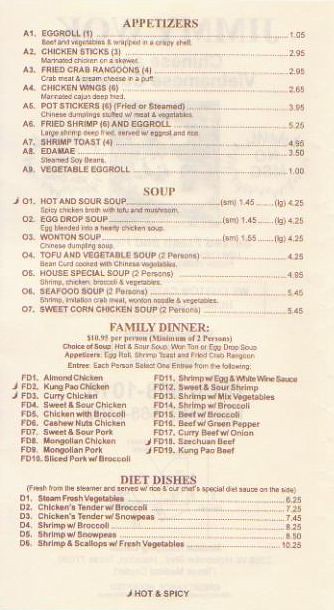Chinese Restaurant Menu (Backside)

**Appetizers**
A1. Egg Roll - $2.50
A2. Chicken Sticks - $3.00
A3. Crab Rangoons - $3.50
A4. Chicken Wings - $4.25
A5. Pot Stickers (Fried or Steamed) - $4.50
A6. Fried Shrimp and Egg Roll - $5.00
A7. Shrimp Toast - $3.75
A8. Vegetable Egg Roll - $2.50
A9. Honey Chicken - $5.95

**Soups**
S1. Hot and Sour Soup - $2.95
S2. Egg Drop Soup - $2.50
S3. Wonton Soup - $3.25
S4. Tofu and Vegetable Soup - $3.75
S5. House Special Soup - $5.25
S6. Seafood Soup - $5.75
S7. Sweet Corn Chicken Soup - $3.50

**Family Dinner**
$10.95 per serving (Minimum of two persons)
Includes:
- Choice of Soup (Hot and Sour, Wonton, or Egg Drop Soup)
- Appetizers: Egg Roll, Shrimp Toast, or Crab Rangoons
- Each person selects one entree from the following:
  - Almond Chicken
  - Kung Pao Chicken
  - Szechuan Chicken
  - Korean Chicken
  - Sweet and Sour Chicken
  - Chicken with Broccoli
  - Cashew Nut Chicken
  - Mingolian Chicken
  - Mingolian Pork
  - Sliced Pork with Broccoli
  - Shrimp with Egg and White Wine Sauce
  - Sweet and Sour Shrimp
  - Shrimp with Vegetables
  - Shrimp with Broccoli
  - Beef with Broccoli
  - Beef with Green Peppers
  - Curry Beef and Onion
  - Kung Pao Beef

**Diet Dishes**
D1. Steamed Fresh Vegetables - $6.95
D2. Chicken Tenders with Broccoli - $7.95
D3. Chicken Tenders with Snow Peas - $7.95
D4. Shrimp with Broccoli - $8.95
D5. Shrimp with Snow Peas - $8.95
D6. Shrimp and Scallop with Fresh Vegetables - $9.95

Prices for all items are listed next to the respective dish.